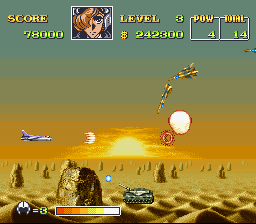The image depicts a classic, vintage-style arcade game set in a desert landscape at sunset. The sandy terrain is dotted with dunes and rolling hills, creating a rugged backdrop for the action. 

In the foreground, a military tank occupies the center-bottom of the screen, suggesting the player's vehicle. Flanking the tank are two aircraft: one on the left-hand side and another on the right-hand side, indicating an aerial component to the gameplay. 

At the top of the screen, essential game information is displayed. On the left, the player’s score is prominently featured, reading 78,000 points, alongside a cartoony image of a pilot, implying the game's military theme. The level indicator shows the player is currently on level 3, and the in-game currency or resources total $242,300.

On the top right, two small rectangular boxes provide additional details: one labeled "POW" lists a count of 4, and the other labeled "Total" shows a count of 14, likely indicating prisoners of war rescued or enemies defeated. 

The combination of nostalgic pixel graphics and military-themed elements creates an immersive, retro gaming experience.